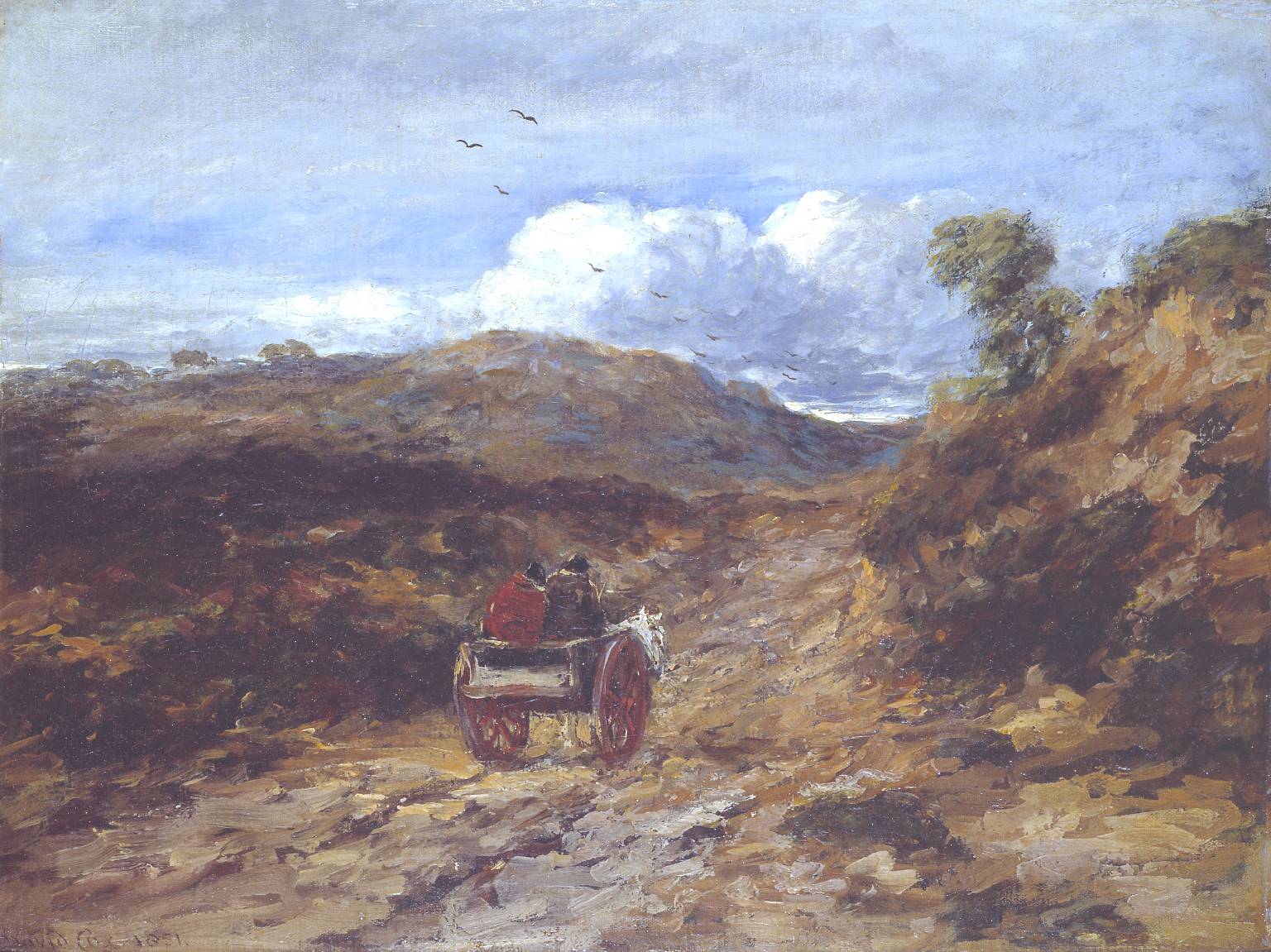In this impressionistic-style oil painting, every brushstroke brings vivid detail to the scene. A white horse pulls a distinctive red-wheeled carriage carrying two figures garbed in red and brown. They traverse a rocky, undulating path through a valley characterized by various shades of brown, flanked by two imposing hills. To the right, a tall green tree stands prominently, while to the left, there are indistinct forms—possibly additional trees or animals—just above the hills. The sky overhead is a serene blue, dotted with fluffy white clouds and birds soaring above, creating a harmonious and vibrant tableau.